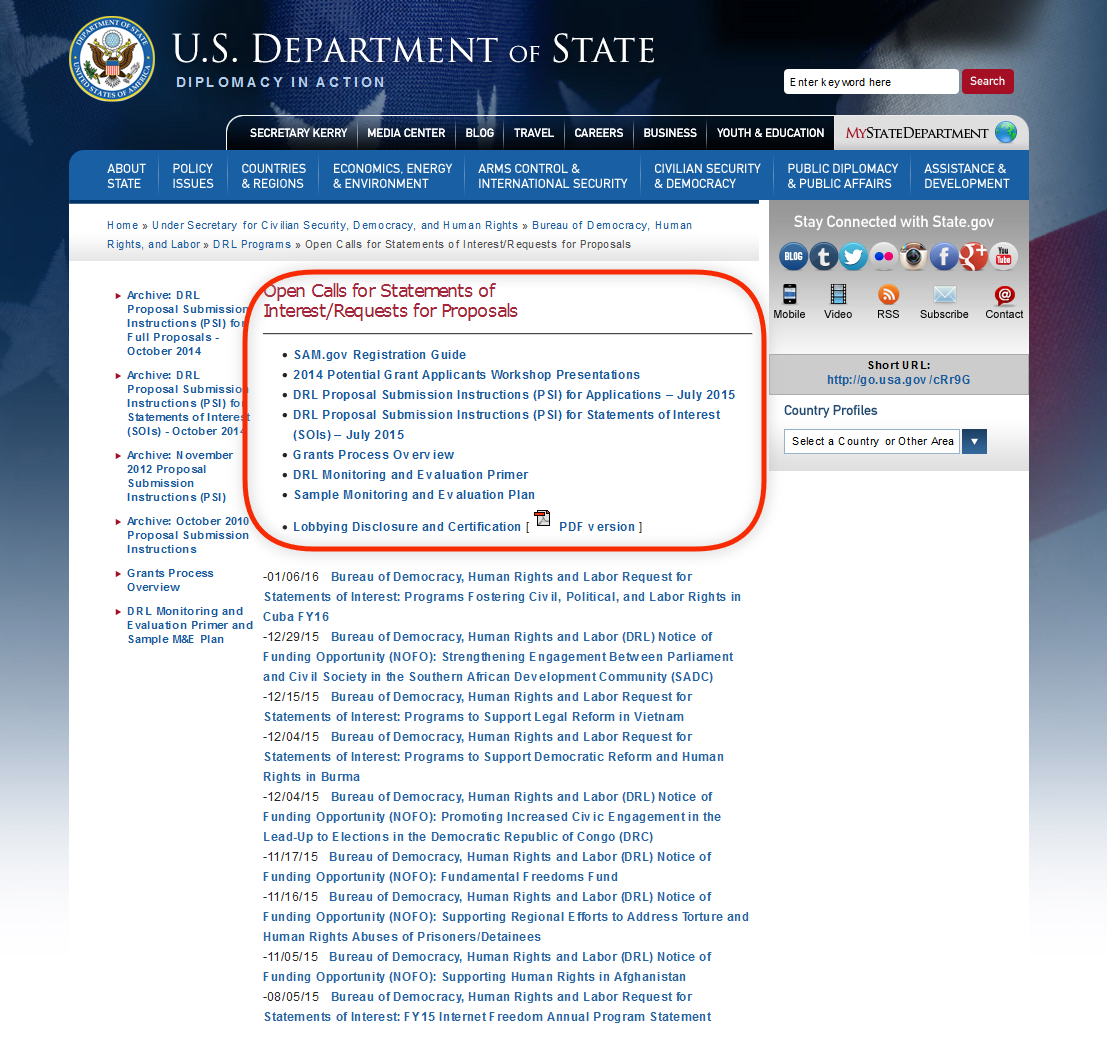The image features the U.S. State Department's website, presented in a portrait orientation, fading gradually towards the bottom. The backdrop is an American flag with a vanishing gradient that transitions to white as it descends, while the upper portion remains distinctly blue, displaying a few stars. Dominating the header is the American crest, accompanied by the text "U.S. Department of State, Diplomacy in Action."

The navigation bar includes tabs such as "Secretary Kerry," which indicates the webpage is from the Obama administration era, along with "Media Center," "Blog," "Travel," "Careers," "Business," "Youth and Education," and "My State Department." Below this primary navigation, an additional set of blue tabs offers further navigation to sections like "About State Policy Issues" and "Countries and Regions," with archived documents listed on the left side.

Central to the image is a red box with rounded corners, prominently titled "Open Calls for Statements of Interest / Request for Proposal" in red font. This section highlights various documents essential for individuals seeking guidelines and necessary forms to submit proposals related to the State Department's activities.